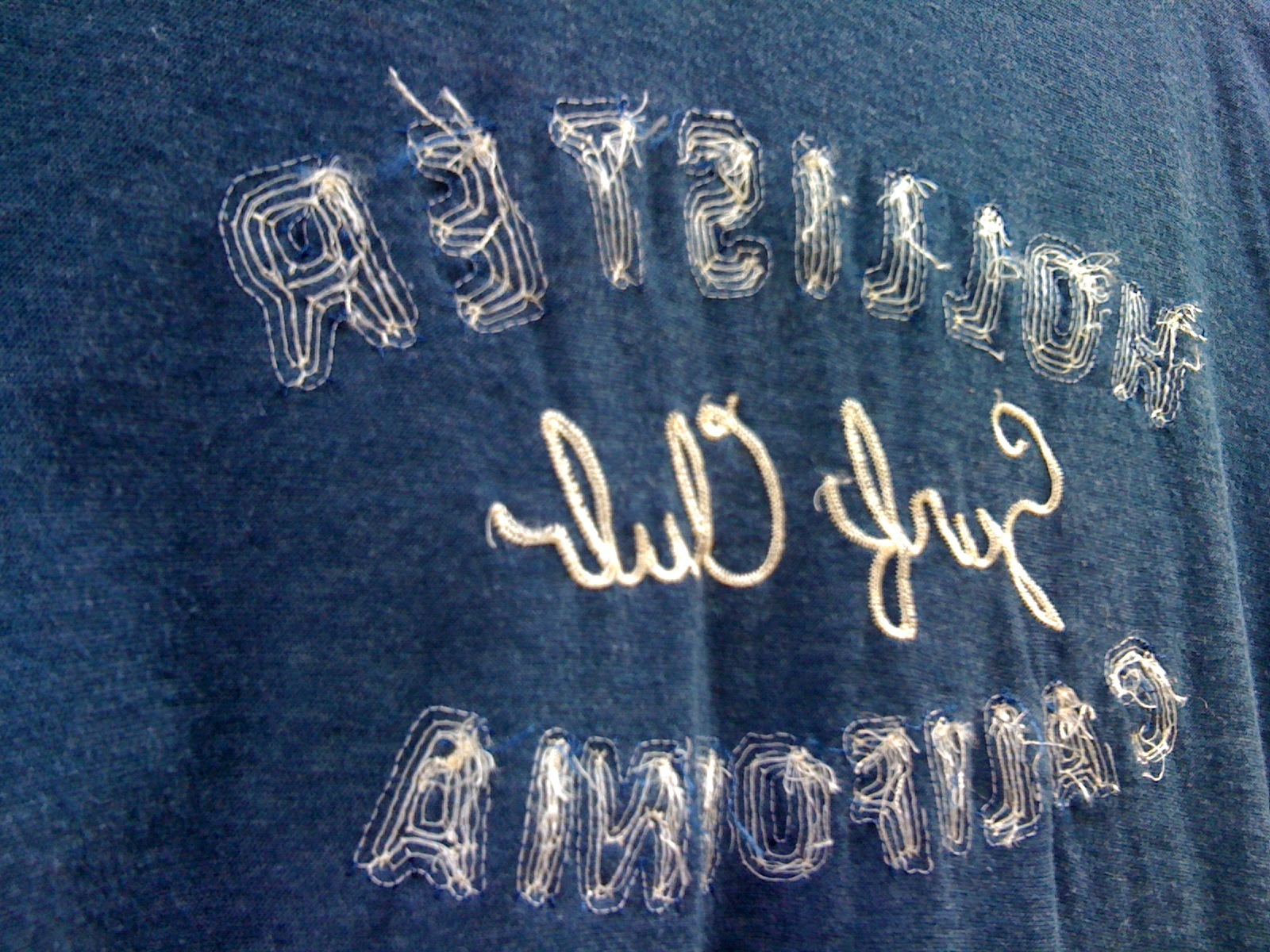A landscape-oriented photograph features a medium blue sweatshirt turned inside-out. Stitched onto the sweatshirt are the words "Hollister," "Surf Club," and "California," all appearing in reverse due to the inside-out orientation. The word "Hollister" and "California" showcase a multi-line design for each character, while "Surf Club" is presented in a solid calligraphy font centered between them. The detailed embroidery and the unique wording style are clearly visible despite the reversed text.